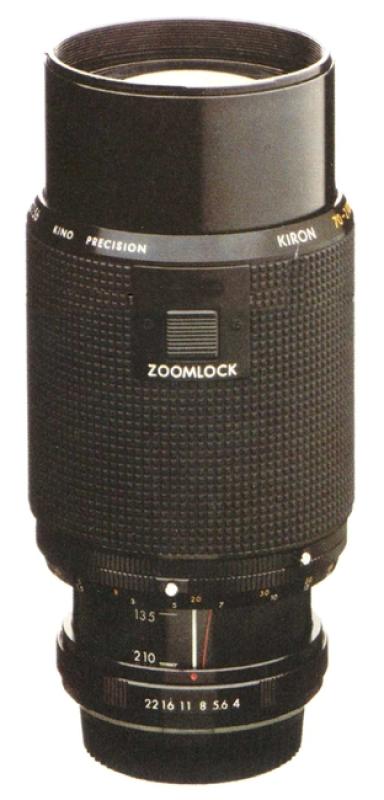This image features an old-school, large telephoto camera lens set against a white background. The overall appearance is slightly grainy and blurry, suggesting that the image might be dated. The lens is cylindrical and takes up the entirety of the image, showcasing its detailed structure. At the top, the lens reveals its internal threads, indicating how it would be attached to a camera body.

The lens exterior is predominantly black, with various sections exhibiting different textures for improved grip. The lens has a glossy, smooth surface at the top, leading into a middle section characterized by a pattern of small black squares, providing a textured grip. Prominently, this middle segment features a button labeled "zoom lock," and above it, white text reads "Kino Precision" and "Curon."

The section below the zoom lock button shows a knurled dial that is likely involved in adjusting the lens settings. Here, marked numbers include the focal lengths 135-210mm. A lower portion of the lens displays engraved f-stop numbers such as 22, 16, 11, 8, 5.6, and 4, indicating its aperture settings. Further down, another textured segment allows additional grip for potential adjustments. Throughout the lens, various dials and markings are visible, contributing to its functional complexity.

Overall, this detailed depiction emphasizes the lens's vintage design and functionality, highlighting its multiple grip sections, labeled buttons, and intricate dial settings.